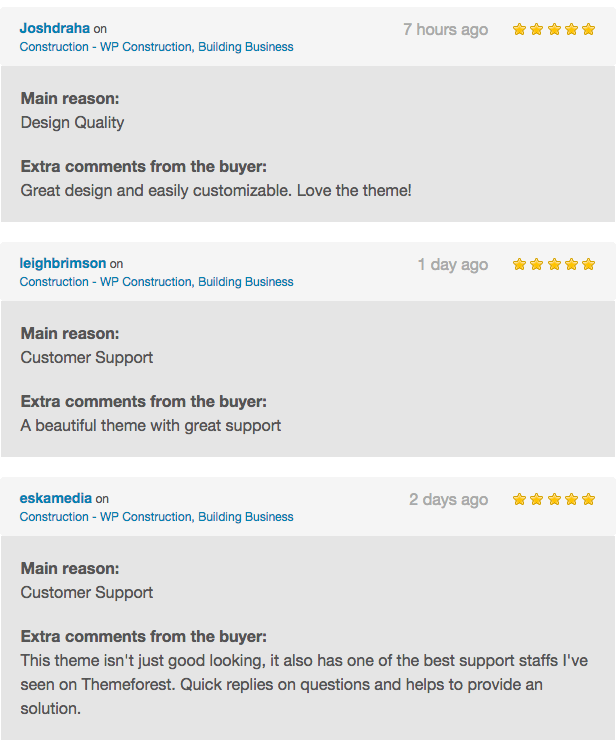Here are the cleaned-up, detailed captions based on the provided information:

---

**Image Caption: Detailed Testimonials for Construction-WP Theme**

- **Top Left:**
  - **Reviewer:** Josh Grahna
  - **Date:** Seven hours ago
  - **Rating:** ★★★★★
  - **Comments:**
    - **Main reasons described:** Design quality
    - **Extra comments from buyer:** "Great design and easy to customize. Love the theme."
  - **Color Scheme:** Blue, black, gray, yellow, light gray, dark gray, and white

- **Middle:**
  - **Reviewer:** Leah Brimson
  - **Date:** One day ago
  - **Rating:** ★★★★★
  - **Comments:**
    - **Main reasons described:** Customer support
    - **Extra comments from buyer:** "A beautiful theme with great support."
  - **Color Scheme:** Blue, black, gray, yellow, light gray, dark gray, and white

- **Bottom:**
  - **Reviewer:** Eskamedia
  - **Date:** Two days ago
  - **Rating:** ★★★★★
  - **Comments:**
    - **Main reasons described:** Customer support
    - **Extra comments from buyer:** "This theme isn’t just good-looking, it also has one of the best support staffs I’ve seen on ThemeForest. Quick replies on questions and helps to provide solutions."
  - **Color Scheme:** Blue, black, gray, yellow, light gray, dark gray, and white